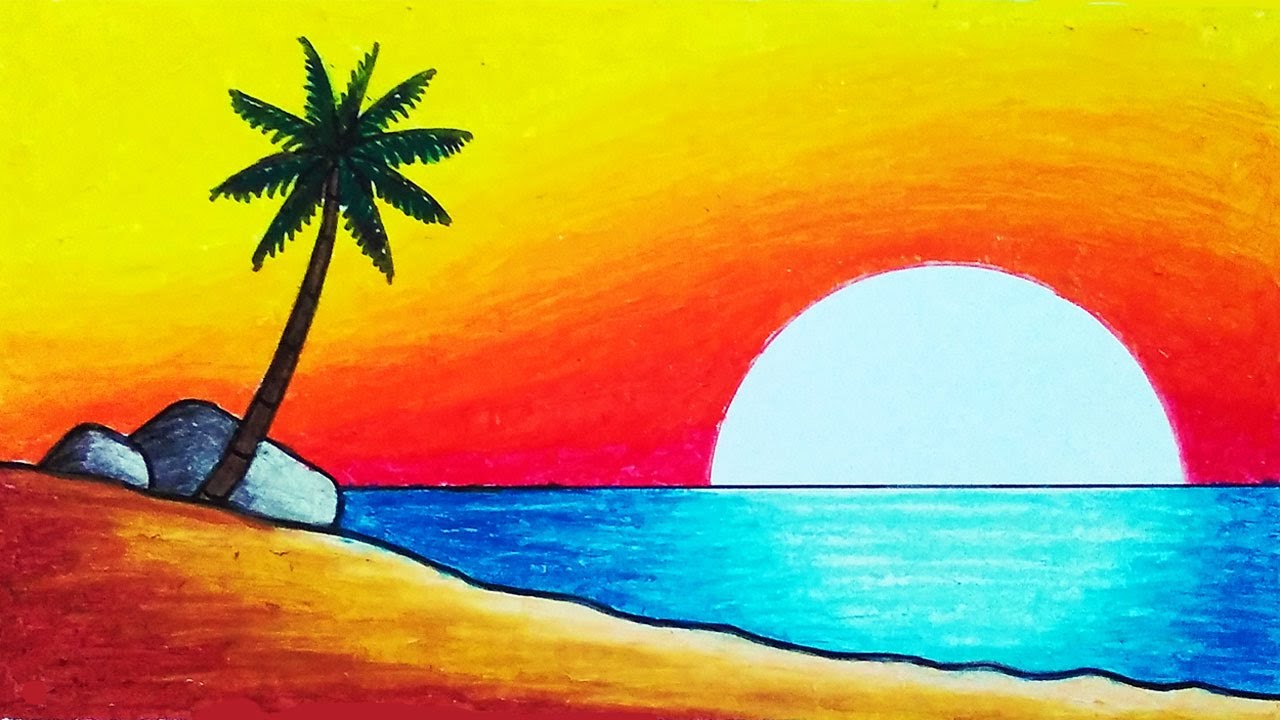This is a detailed and colorful scene depicting a sunset over an island beach, created with what appears to be colored pencils or possibly crayons. The rectangular image, approximately five to six inches wide and three inches high, showcases a striking contrast of hues. At the center of the composition is a large, white sun partially dipping into the horizon, casting its glow over a rich blue sea. The water near the sun transitions to a lighter blue, portraying the brightness of the setting sun.

Surrounding the sun, the sky is alive with vibrant reds and yellows, blending subtly to imply shades of orange without actually depicting it. This atmospheric gradient stretches upwards from a dense, dark orange band to lighter yellows across the sky. Below, the beach itself features a gradient from reddish-brown to lighter tan colors, with a bold black outline marking the island’s edge.

Dominating the island is a single palm tree, its dark brown trunk and green leaves standing tall against the colorful backdrop. Nestled around the base of the palm are two gray boulders, adding texture to the scene. The entire composition is infused with a bright and lively energy, capturing the serene beauty of a beach at sunset.